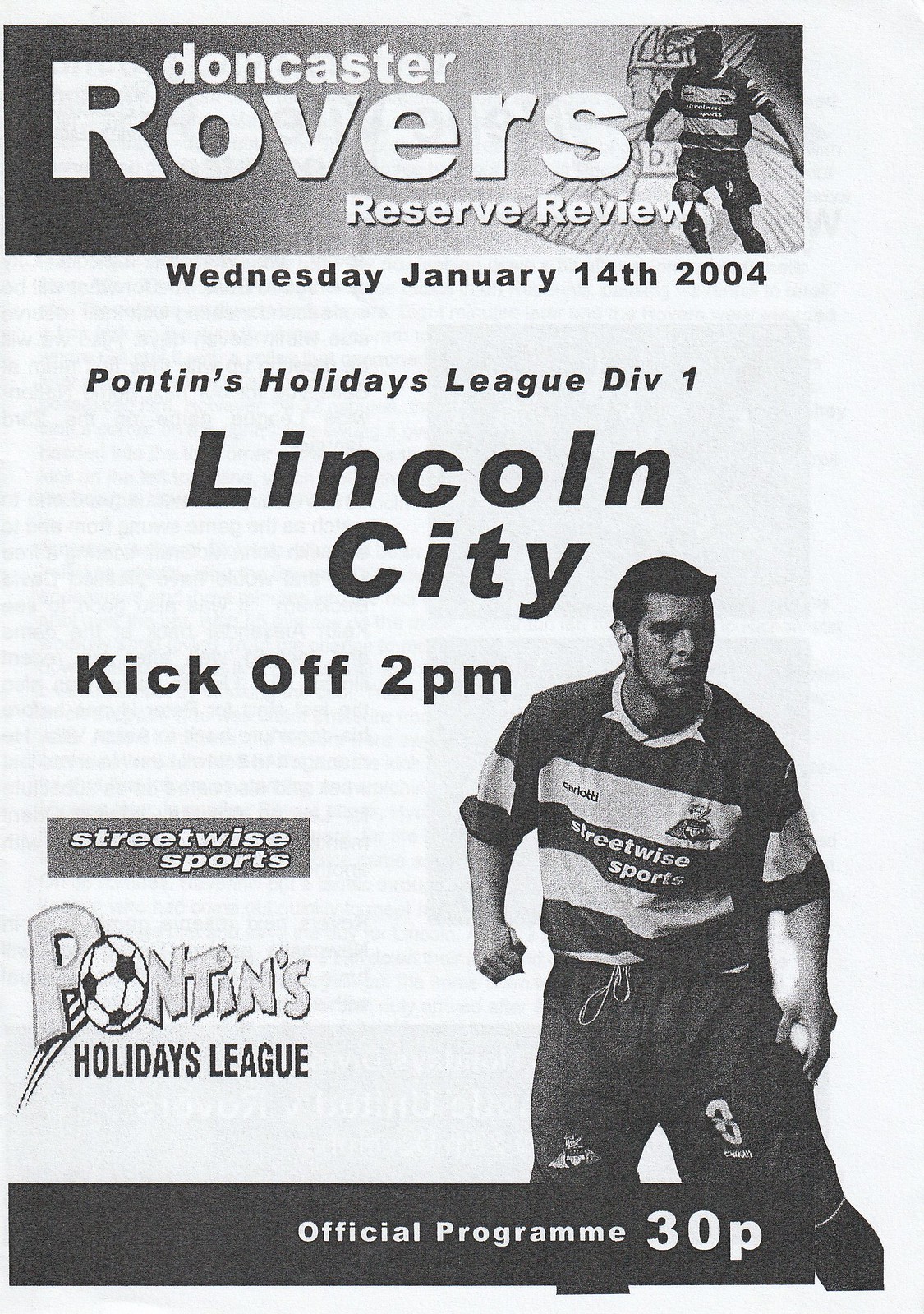The official program for 30P is a black and white poster from January 14, 2004, featuring the "Doncaster Rovers Reserve Review" at the top. The date, Wednesday, January 14th, 2004, is printed prominently beneath the title, followed by the event details: "Pontins Holiday League Division 1, Lincoln City, kickoff 2 p.m." The design includes a black and white image of a soccer player wearing a "Streetwise Sports" jersey and shorts, positioned to the right. The poster features two logos: "Streetwise Sports" and "Pontins Holiday League," the latter with a soccer ball as the 'O' in Pontins. Despite the image's modern date, the black and white photocopied quality lends an older, cranny appearance to the artwork.